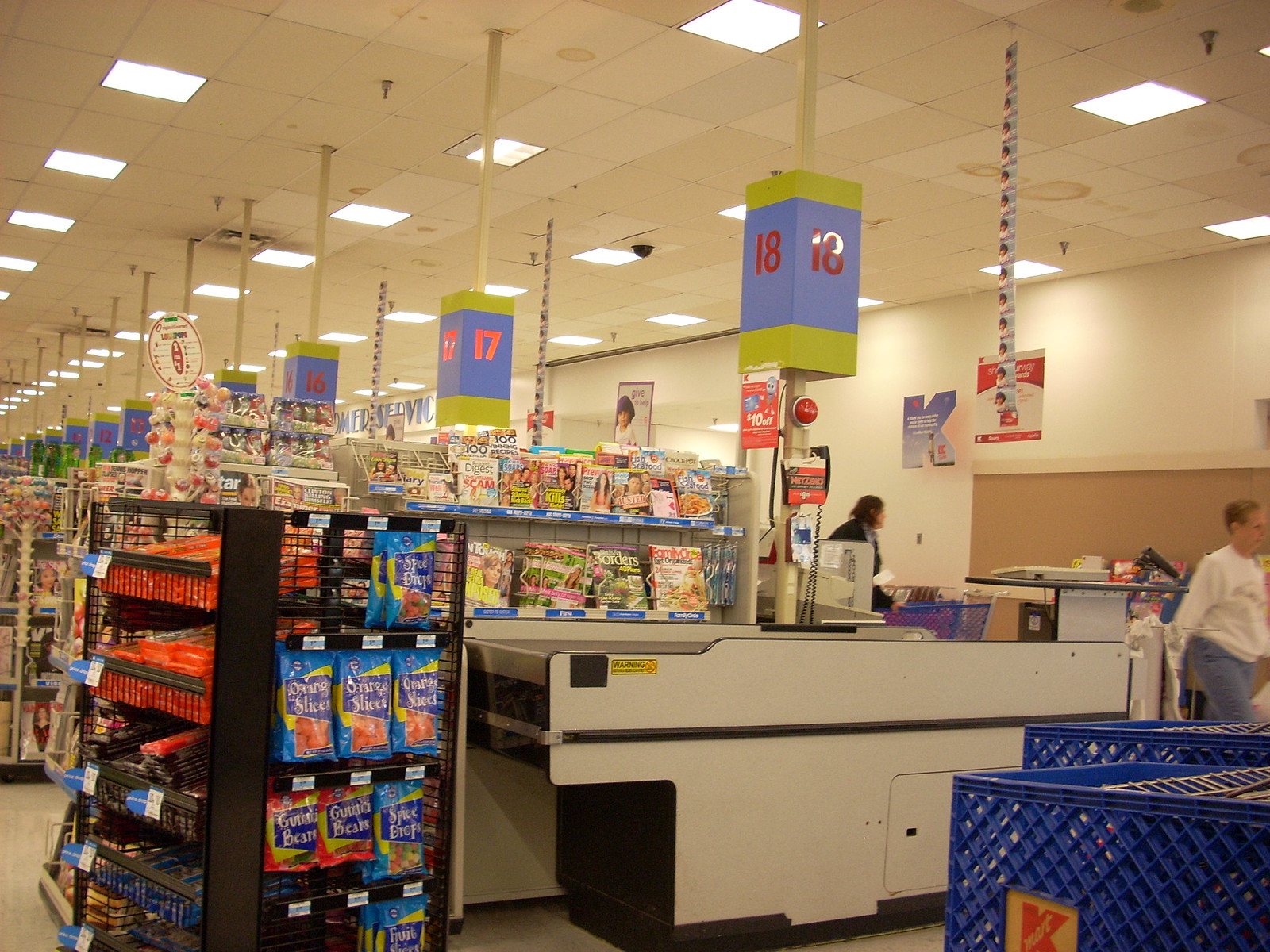The image depicts the interior of a Kmart store featuring a distinctly tiled ceiling adorned with numerous light fixtures. In the bottom right corner, there are two blue Kmart shopping carts. To the left of the carts is a conveyor belt at a checkout station, with shelves of various items including magazines, blue and red bags, and candy. In the background, a person with short hair, wearing a white shirt and blue pants, is walking past a white wall emblazoned with a large red 'K'. Multiple promotional pictures hang from the ceiling, and checkout lanes 16, 17, and 18 are visible, with lane 17 indicated as open. More shelves stocked with snacks and goodies are visible throughout the store.